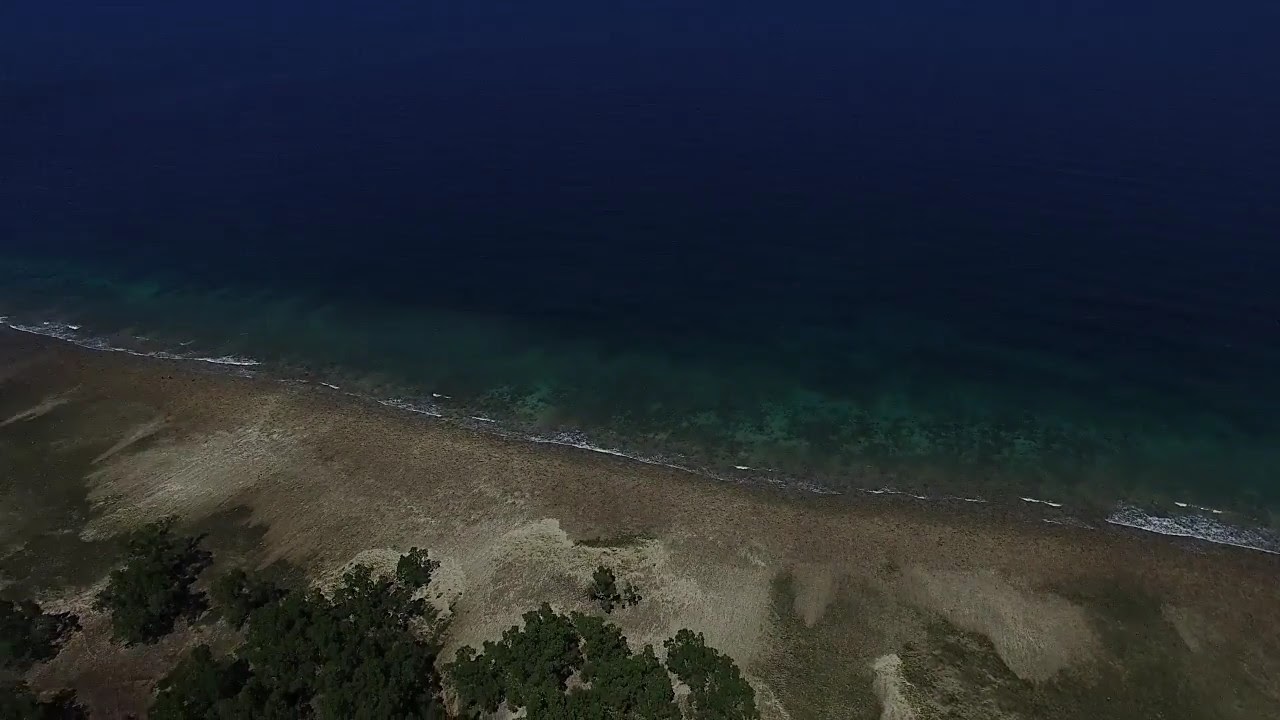The photograph captures a serene, natural shoreline, viewed from an elevated perspective, possibly from a cliff or an aerial vantage point such as a plane or helicopter. The top portion of the image is dominated by the deep, dark blue expanse of the ocean, transitioning into a lighter blue-green hue as it approaches the shore, revealing patches of coral or seaweed beneath the surface. White-capped waves indicate where the water breaks over a sandbar. This sandbar, initially dark from the receding tide, transitions into a lighter, dry sandy area closer to the beach.

The shoreline itself is a mottled brown, untouched by human presence or infrastructure, lending it a completely deserted and natural appearance. Driftwood or sea algae is scattered across the beach, particularly on the left and central parts, diminishing towards the right. The landscape extends into green shrubs and trees, creating a lush border against the pristine sand. The entire scene is shrouded in dim light, suggesting it might be taken during a darker hour, contributing to the image's tranquil yet slightly mysterious atmosphere.